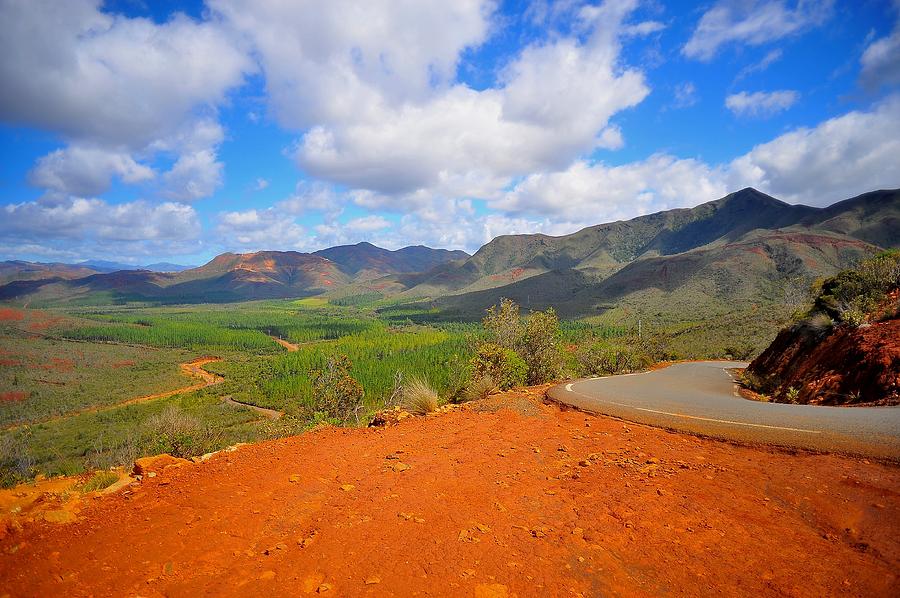This detailed photograph captures a vast daytime landscape under a dynamic sky filled with large white and gray clouds set against a dark blue backdrop, accented with cyan in the lower left corner. A majestic range of mountains stretches across the middle of the image, revealing a rich tapestry of colors—green and brown hues dominate, while the leftmost mountain sports dark blue with brown accents. As the eye moves right, the mountains transition to a lighter olive green with splotches of brown, with the farthest right peak casting a shadow, giving it a dark blue appearance. 

In the foreground, a lush green pasture dotted with patches of lighter grass extends toward the background, intersected by a small dirt path that meanders toward the lower left corner. To the right of this path, small brown and yellow-accented bushes add texture to the scene, alongside a patch of orange and brown clay embedded with lighter rocks. A narrow gray paved road with white markings runs along this area, leading to a pile of brown and orange rocks crowned with dark green foliage, situated at the center-right of the image. The lower section of the image features crumbled stones and pebbles scattered across the coppery soil, enhancing the rich, earthy foreground. The entire scene extends into the background, where lofty mountains with lighter grass and brown dirt crowns rise, encapsulated by the vibrant, cloud-filled sky.